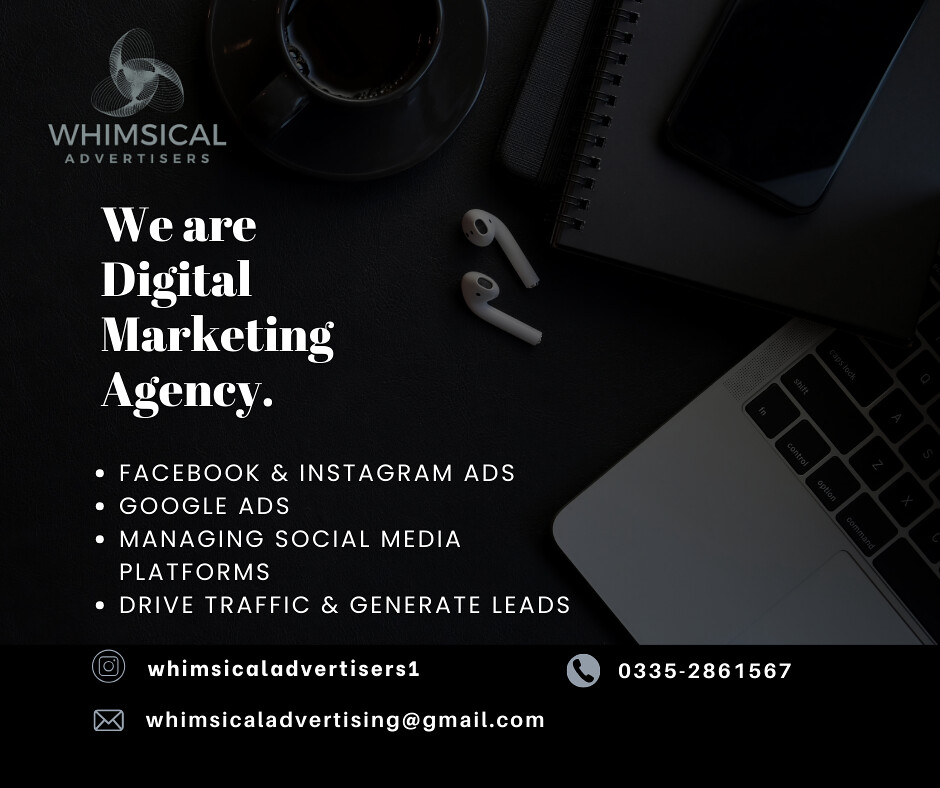The image appears to be a promotional banner from Whimsical Advertisers, a digital marketing agency. With a dark, black background, the top left corner prominently features the company's name, "Whimsical Advertisers," and the tagline "We are a digital marketing agency" in white text. The image captures the edge of a MacBook, showcasing part of the keyboard and screen, along with wireless AirPods placed nearby. Additionally, a cup of coffee on a saucer and a notebook with a phone on top are seen in the frame, lending a workspace vibe to the setting. Highlighted services such as Facebook and Instagram ads, Google ads, social media platform management, driving traffic, and generating leads are listed with bullet points. Contact details include an Instagram handle "Whimsical Advertisers 1," an email address "WhimsicalAdvertising@gmail.com," and a phone number "0335-286-1567," displayed with respective icons.